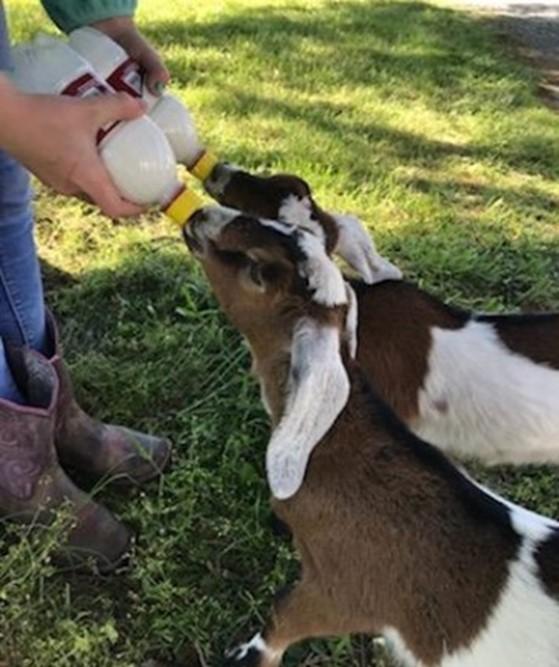In a grainy photograph, two brown and white spotted goats with long white ears and white caps on their heads angle their heads upward to drink from two plastic bottles with yellow caps, seemingly filled with milk. The bottles are held by two hands, one of which has an olive green painted nail and is clad in an olive green sleeve. Only a portion of the bottle-holder is visible in the left side of the frame, revealing blue jeans and subtly pinkish red cowboy boots standing in slightly overgrown grass. The scene suggests a rural atmosphere, possibly during daytime, as careful attention is given to feeding the goats amidst a natural grassy setting.